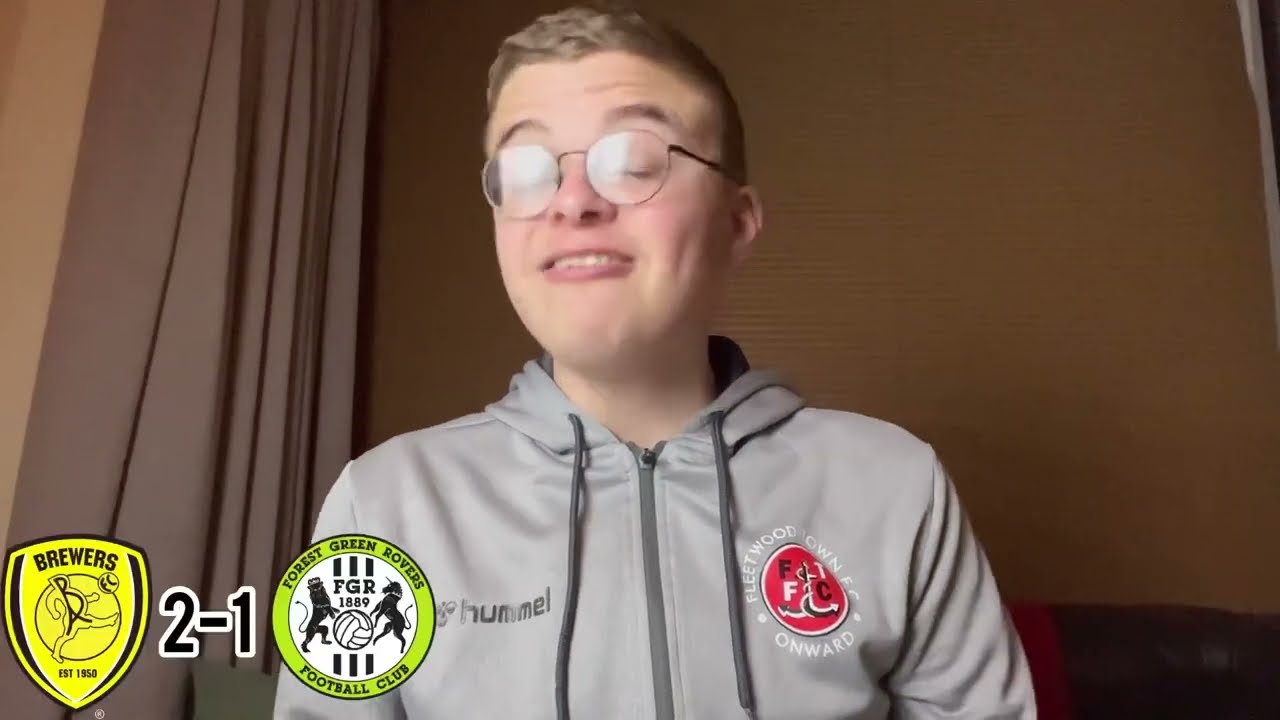This image depicts a young man, likely a teenager around 15 to 17 years old, standing indoors, possibly in his house. He has short, light brown hair and is wearing round glasses. His eyes are closed and his mouth is open mid-speech, showing the top row of his teeth. He is dressed in a long-sleeved gray hoodie jacket that features two prominent logos: on the right side, there is a Fleetwood Town F.C. emblem that includes the phrases "Fleetwood Town Onward" and "FTFC" inside a red circle with white and black ship anchors; and on the left side, there is the black logo of Hummel. Behind him, there is a brown wall and a heavily pleated brown curtain. In the top left corner, part of a light beige wall is visible. The bottom left corner of the image shows a scoreboard from a soccer match, indicating a score of 2-1 with the Brewers leading. The Brewers' shield-shaped logo is yellow with black text and features the letters "B" and "A" forming the image of a man kicking a ball, alongside the text "Established 1950." Adjacent to this is the round emblem of Forest Green Rovers Football Club, showcasing a green border, white and black text, and a central design of a lion wearing a crown, a unicorn, and a soccer ball labeled "FGR 1889."